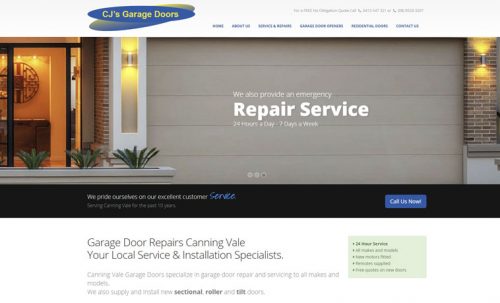The image depicts a computer screenshot of a website dedicated to garage door services. Dominating the layout is a large horizontal rectangle featuring a photograph of a house with a prominent gray garage door. Flanking the garage door on the left is the main door of the house, accompanied by exterior lights and some neatly trimmed plants. 

Centrally displayed on the garage door is an inscription: "We also provide an emergency repair service 24 hours a day, 7 days a week." Above this image, positioned on the left side, is a large blue oval containing the text "CJ's Garage Doors."

Just beneath the oval, a navigation bar offers clickable options for various sections of the website, including "Home," "Garage Door Services," and "Contact Us."

Below the main image, a headline in bold black text reads: "Garage Door Repairs Canning Vale, your local service and installation specialists." Smaller black text underneath provides additional information, describing the company's specialization in repairing and servicing garage doors of all makes and models in the Canning Vale area, although the text is difficult to read due to its size.

In the bottom right-hand corner of the screenshot, there is a tiny green box with text that is too small to decipher clearly.